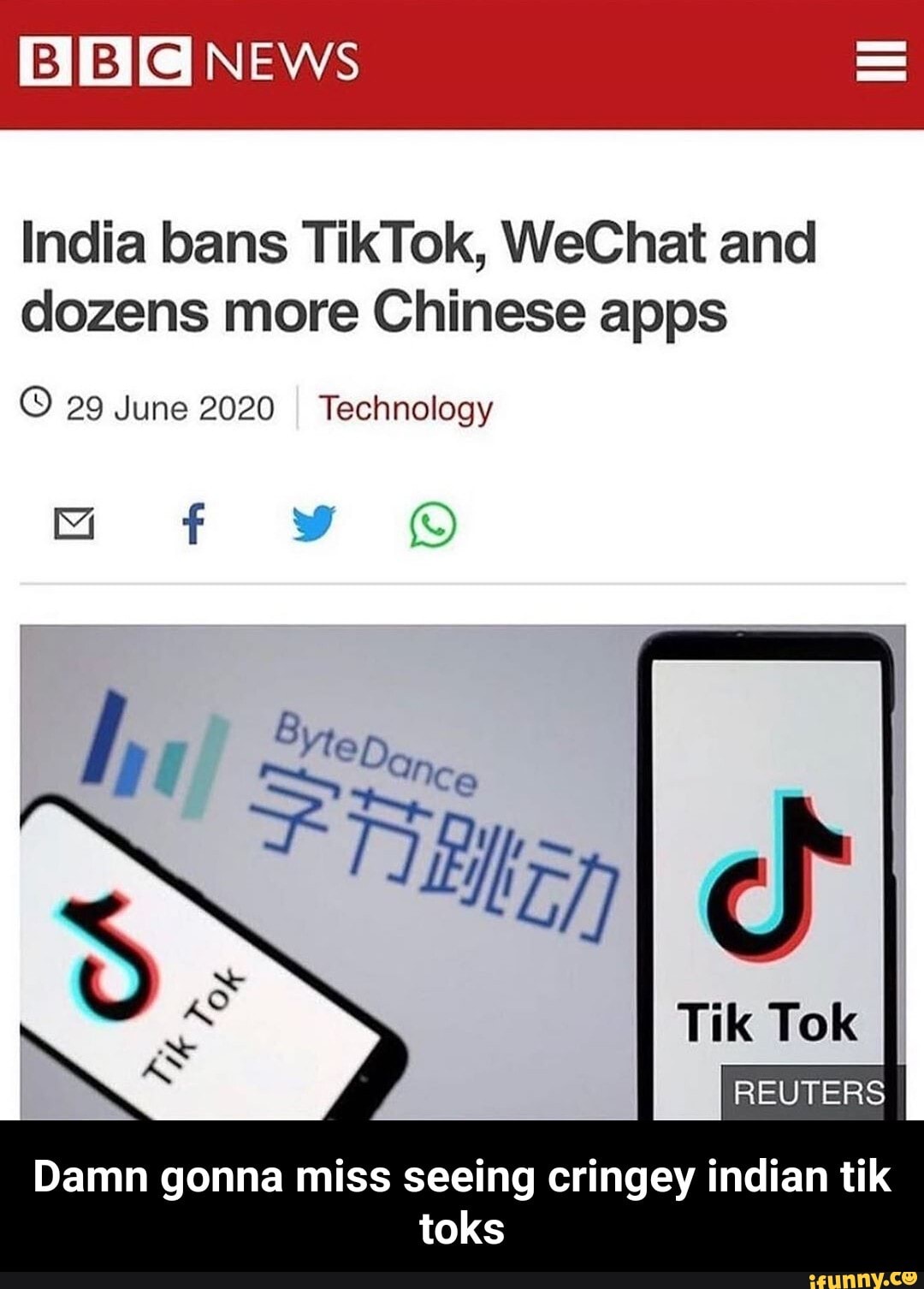The image features a prominent red band across the top with the text "BBC News" in white. The letters 'B', 'B', and 'C' are each placed within white boxes, through which the red background is visible. On the right side of the red band, there is a menu icon consisting of three horizontal bars.

Below the red band, on a white background, the headline "India bans TikTok, WeChat, and dozen more Chinese apps" is prominently displayed, followed by the date "29 June 2020" and the category "Technology." Below this text, a series of icons representing an envelope, Facebook, Twitter, and WhatsApp are lined up.

A gray line separates the header section from the main image below it, which showcases several smartphones displaying the TikTok logo prominently on their screens. The background of the image is light gray, featuring the text "ByteDance" in stylized blue font, with both 'B' and 'D' capitalized. Beneath this text, there is Chinese or Japanese kanji script also in blue. Adjacent to the text are vertical bars in varying shades of dark blue, light blue, medium blue, medium green, and light green.

At the bottom of the image, the words "Damn gonna miss seeing cringy Indian TikToks" are written in black. Finally, in the bottom right corner, the watermark "ifunny.co" appears in yellow.